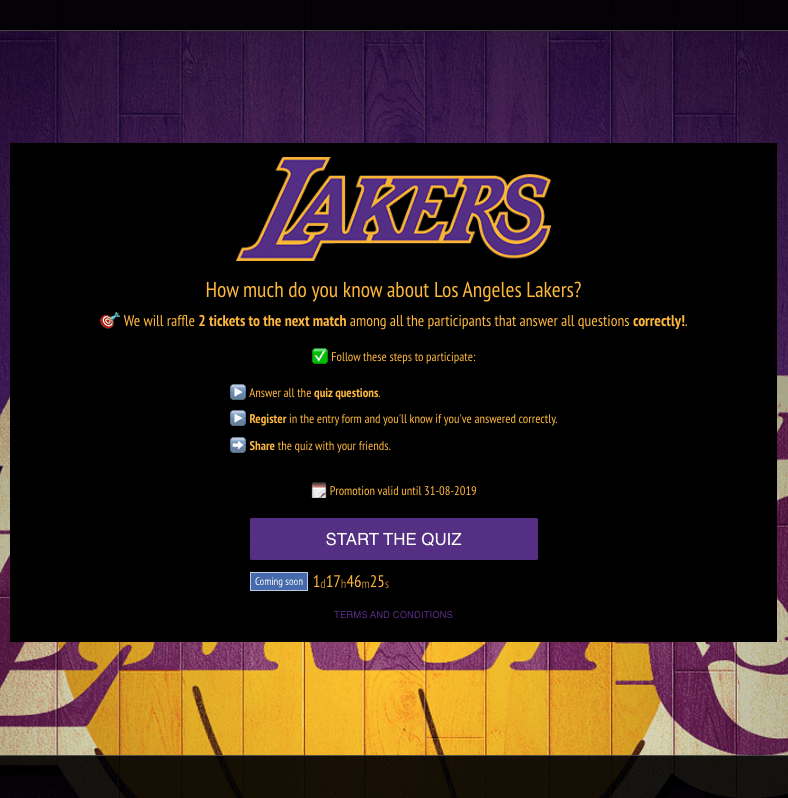This is a detailed webpage for a quiz about the Los Angeles Lakers, designed with the team's iconic purple and gold colors. The title "How Much Do You Know About Los Angeles Lakers?" is prominently displayed. Below this, a bullseye graphic with a dart in it encourages participation by mentioning a raffle: "We will raffle two tickets to the next match among all participants that answer all questions correctly!" A green box with a white checkmark provides instructions: "Follow these steps to participate."

The steps are listed vertically with right-facing arrows:
1. Answer all the quiz questions.
2. Register in the entry form.
3. Share the quiz with your friends.

On the right side, there is a note stating, "Promotion valid until 30/08/2019," next to a square text box. Further down, a purple button labeled "Start the Quiz" invites users to begin, while another rectangular box displays a countdown timer: "1 day, 17 hours, 46 minutes, and 25 seconds." The page also includes a tab for "Terms and Conditions."

Finally, the clear call to action rounds off this interactive and engaging Lakers trivia quiz.